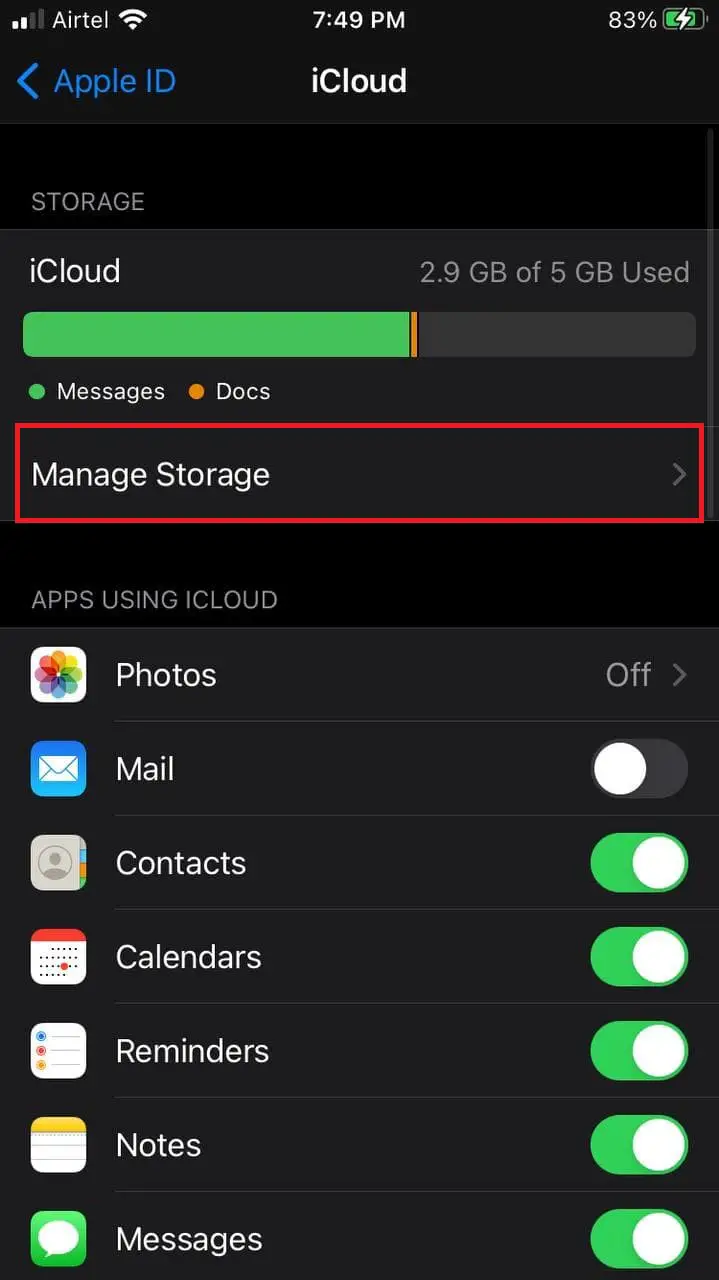An informative screenshot from an iPhone displays various details regarding the device's status and iCloud settings. The device is connected to the Airtel network, showing two out of four cellular signal bars. A fully connected Wi-Fi signal with three bars is also visible. The time in the top center reads 7:49 p.m., and the battery level on the top right corner is at 83%. Just below the status bar, the screen shows a blue ‘Apple ID’ text with a back button pointing left, and an "iCloud" title centered at the top.

The main section details iCloud storage usage: 2.9 GB out of a total 5 GB is used. A color-coded legend indicates the types of data stored; green represents messages, orange represents documents. Below this, there is a red rectangle enclosing the option to 'Manage Storage'. The subsequent section lists the apps using iCloud. For 'Photos', 'Mail' is toggled off, while 'Contacts', 'Calendars', 'Reminders', 'Notes', and 'Messages' are toggled on, indicating that these apps are currently backed up to iCloud. The background of the screen is predominantly black, with shades of darker gray used for the section listing the apps.